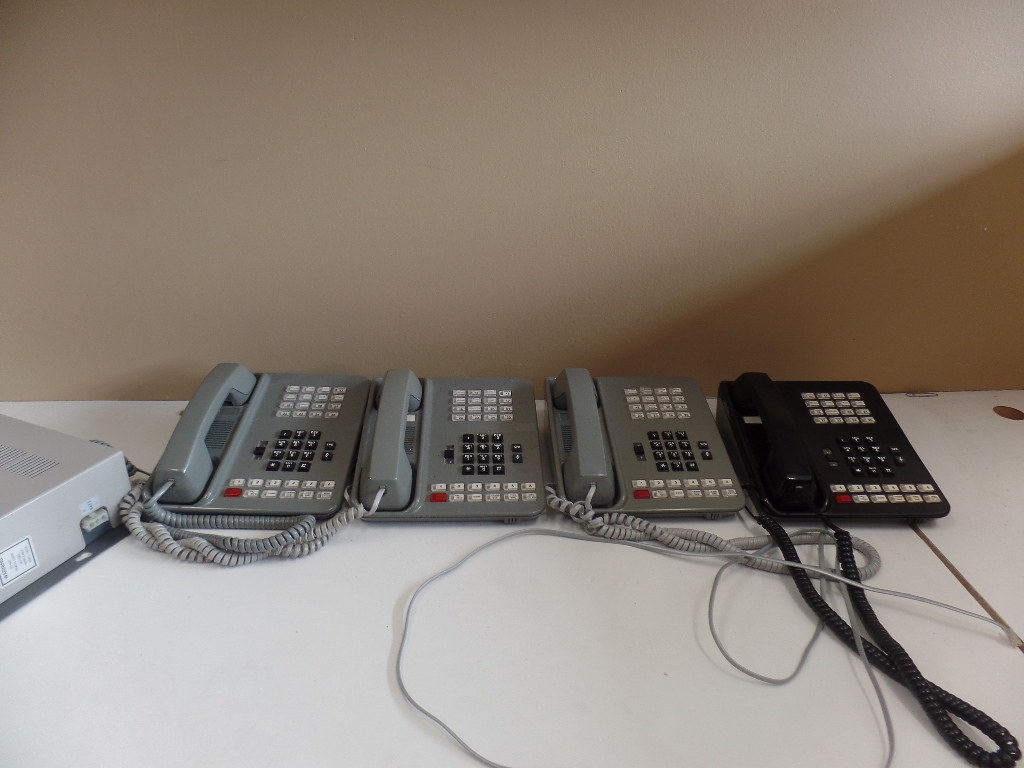This is a photograph of four standard office landline telephones arranged side by side on a white desk in front of a taupe-colored wall. Each phone features a handset on the left side, connected by a long, curly cord, with the right side housing a traditional numeric keypad flanked by numerous additional buttons. These buttons are likely for quick dialing, phone memory, and other functions such as putting calls on hold or transferring them. The phones, reminiscent of those used in offices around the 1990s, include three gray models and one black model. The desk appears to have a hole drilled in it for cord management, reinforcing its role in a business setting.